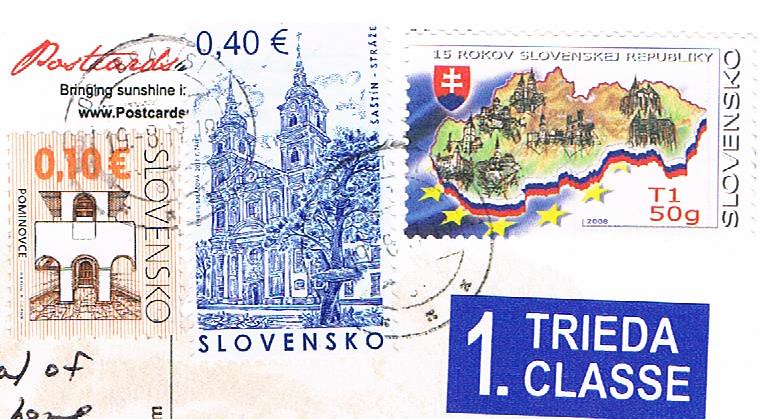This image showcases a postcard adorned with several postage stamps. In the upper left corner, there's a red cursive inscription that reads "postcards." Prominently featured are multiple stamps bearing the name Slovensko, indicating a connection to Slovakia. One stamp, colored blue and white, features an illustration of a tall tower or castle and is marked with "0,40 euros" in the corner. Another stamp, reddish-brown in color, shows the interior of a building with arched walkways and is labeled with "10 cents" or "10 euros". Yet another stamp, displaying a map outline or country silhouette, bears the inscription "15 rokov Slovensko Republiky" and is priced at "15." A blue rectangle on the right side says "1 Trida Klasse," translating to "First Class." Additionally, there is an ink stamp, indicating it has been processed by postal services. The entire image emphasizes the stamps, with almost all visible sections of the postcard covered by them, providing a rich, detailed glimpse into international postage.